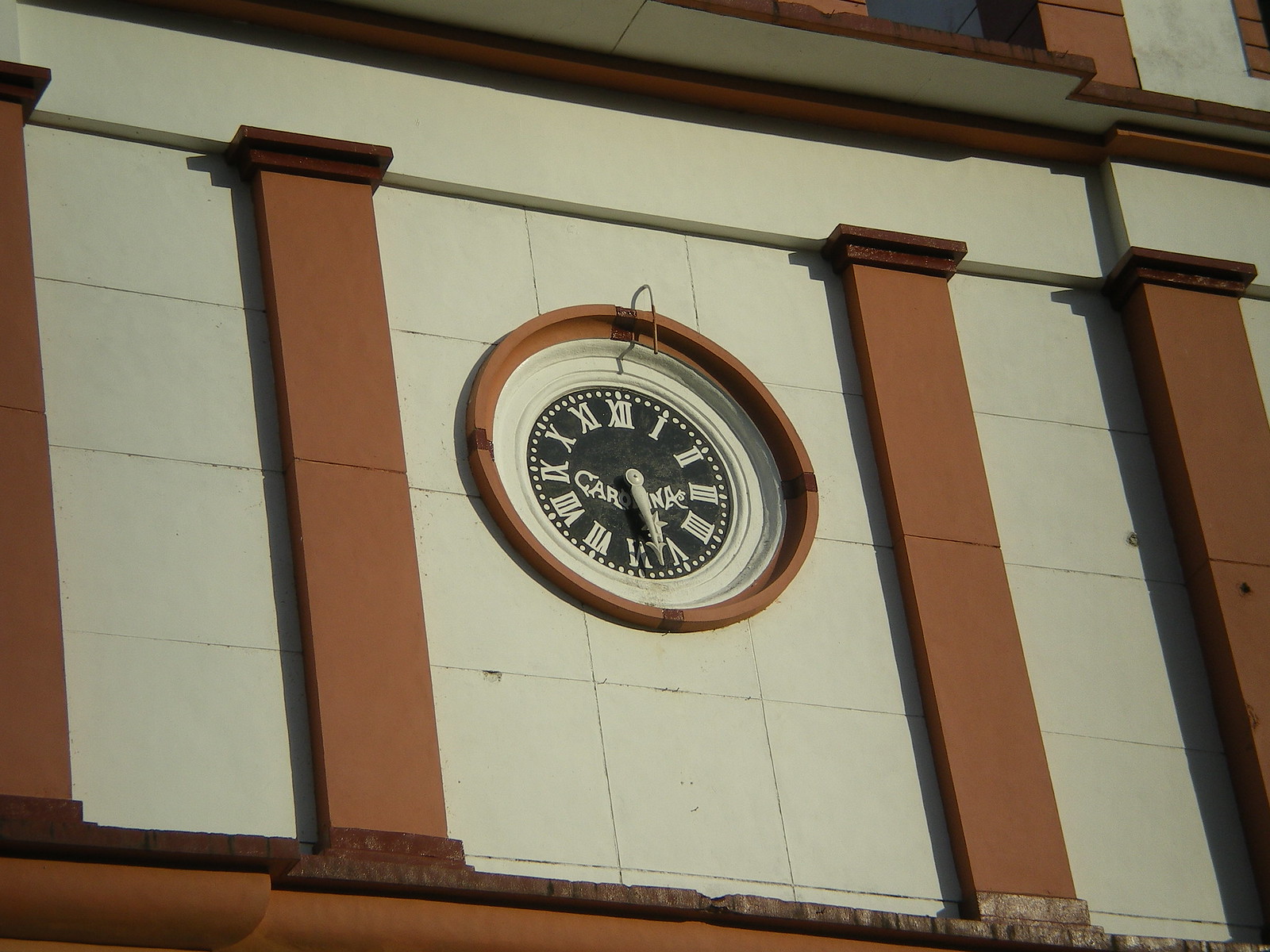In this outdoor color photograph taken during the daytime, the camera captures a close-up, slightly upward-angled view of a grand architectural clock embedded in a city-center building. The image is in landscape orientation, revealing a framed shot of the clock face and a segment of the ornate facade. The building features off-white square blocks arranged in a grid pattern and medium brown, slightly protruding vertical columns composed of rectangular redstone. Central to the image is the analog clock, which is set to 5:30. The clock face itself is black, adorned with white Roman numerals and matching white hands, with the inscription "Carolina" just below the clock hands. Surrounding the black clock face is a white trim bezel, beyond which lie several concentric circles. The innermost circle appears to be made of a beige-y cream-colored stone, while the outermost circumference is terracotta. At the four, three, six, and nine positions, brown strips stretch from the inner to the outermost circumference, adding to the intricate design. The sun illuminates the facade from a high angle, casting light on the elegant and structured exterior.